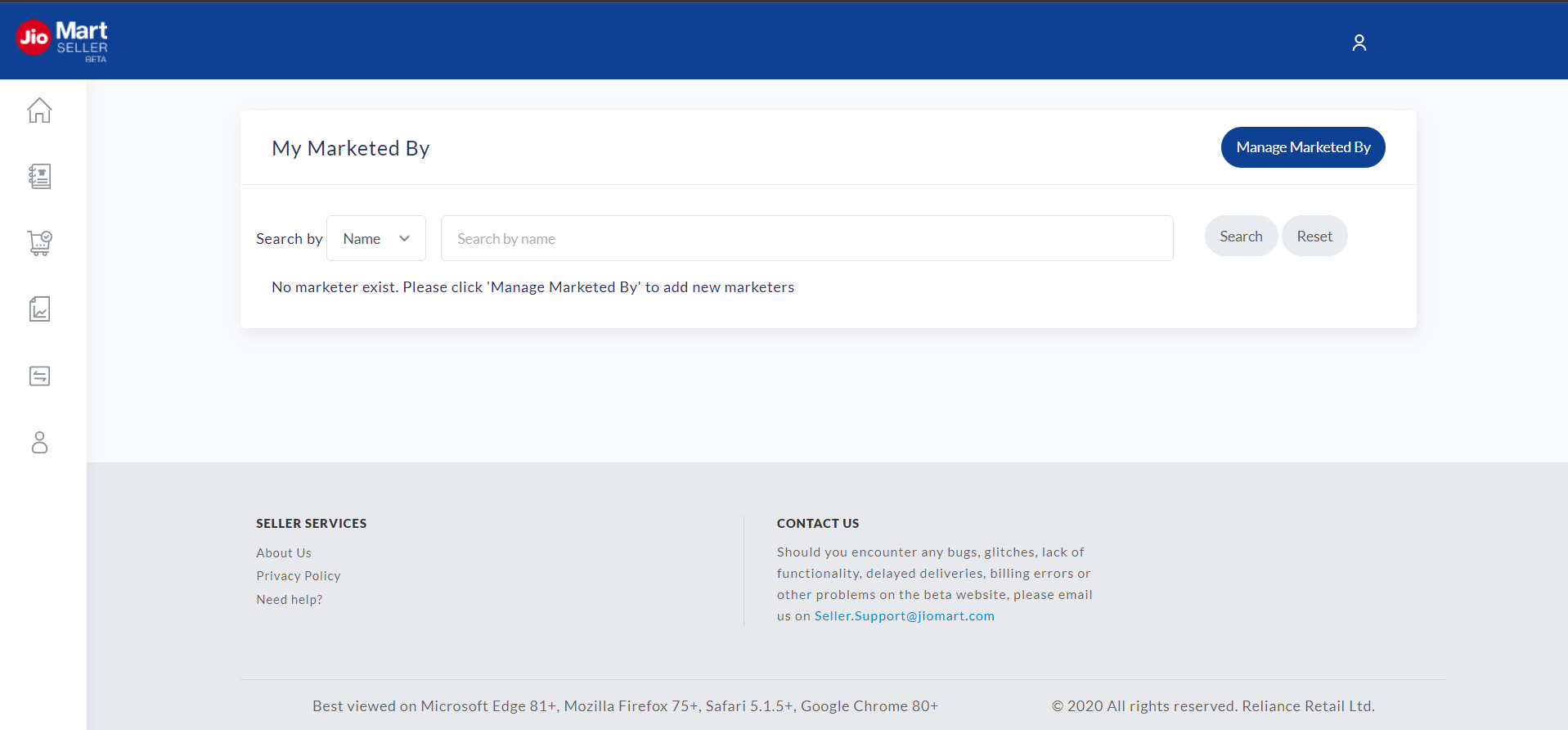The interface features a "JIO" logo in white set on a red circle, with the text "Mart" in white next to it. Below, the word "Seller" is displayed, followed by "AFTA"; all of these elements are situated on the left side. To the right, there is a white person icon.

Below the header, a navigation bar on the left side includes icons representing Home, a notebook, a cart, an Excel spreadsheet, a square with directional lines, and another person icon.

The central part of the screen is dominated by a white pop-up box labeled "My Market Buy". It includes a drop-down menu with the prompt "Search by name", a search field also labeled "Search by Name", and two gray buttons labeled "Search" and "Reset". 

Above this search field is a blue button labeled "Manage Marketed Buy". 

Beneath the search field, a message states, "No Marketer Exists. Please click Manage Marketed Buy to add a new marketer."

The left-hand side features links titled "Seller Services," "About," "Privacy Policy," and "Need Help."

Centered at the bottom, it also says "Contact Us" with a note: "Should you encounter any bugs, glitches, lack of functionality, delays, delayed deliveries, billing errors or other problems on the beta website, please email us at seller.support@jiomart.com."